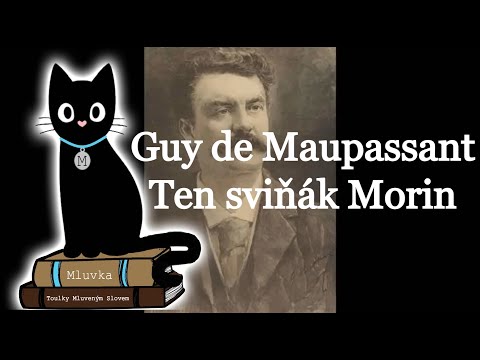The color image merges vintage black-and-white photography with vibrant color illustrations in a landscape orientation. At the center is a detailed and realistic black-and-white portrait of a man, presumed to be Guy de Maupassant, characterized by dark curly hair, a pronounced mustache, and a neutral expression as he gazes slightly upward to the right. He is seen from head to mid-chest, dressed in a dark jacket, shirt, and tie. This photograph, enclosed in a black horizontal rectangle, bears bold white text across the middle that reads "Guy de Maupassant" with a second line below that appears garbled as "10 Sphinox Morin."

Flanking this vintage photograph on the left is a charming and whimsical cartoon illustration of a black cat with wide, white eyes and a pink heart-shaped nose. The cat, adorned with a blue choker and a silver medallion marked with an "M," assumes an upright posture, sitting on its back legs atop a stack of two hardcover books—one beige and one dark brown. The feline gazes directly at the viewer with a curious expression, emphasizing the blend of playful illustration against the formal photographic portrait, all set against a stark black background.